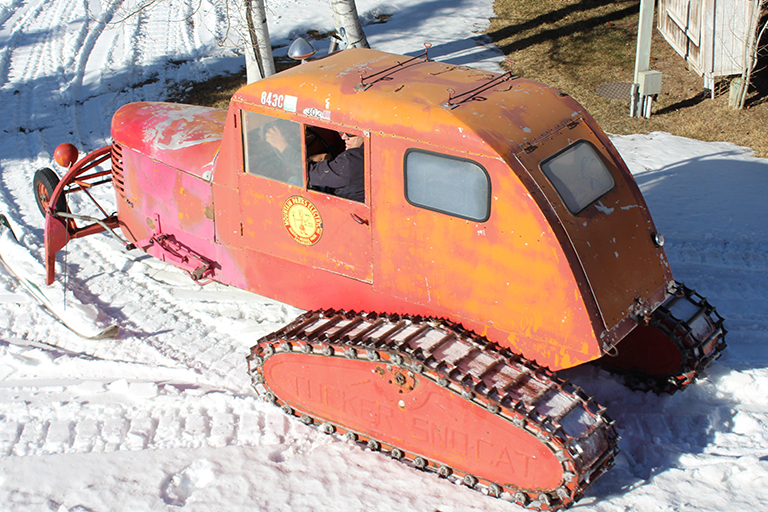In this photograph, an old Tucker Snowcat is navigating a snowy terrain, likely in a rural or farm-like setting. The machine is marked with an 843C designation in the top left corner and features an official sticker on the door. The body of the Snowcat is visibly aged, displaying a mix of rusted, corroded-looking orange, faded red, and pink hues. Its rear has heavy treads similar to those found on a tank, ensuring it can traverse the snowy landscape effectively. The front part includes an engine compartment extending forward, complemented by a complex frame equipped with skis and a small wheel to facilitate smooth movement over the snow. A man wearing sunglasses and a black jacket is seated inside the large, windowed compartment, suggesting space for both driving and additional storage behind him. The machine's unique appearance and specialized structure hint at its use for snow transport, potentially for activities like navigating ski slopes or conducting forest rescues.